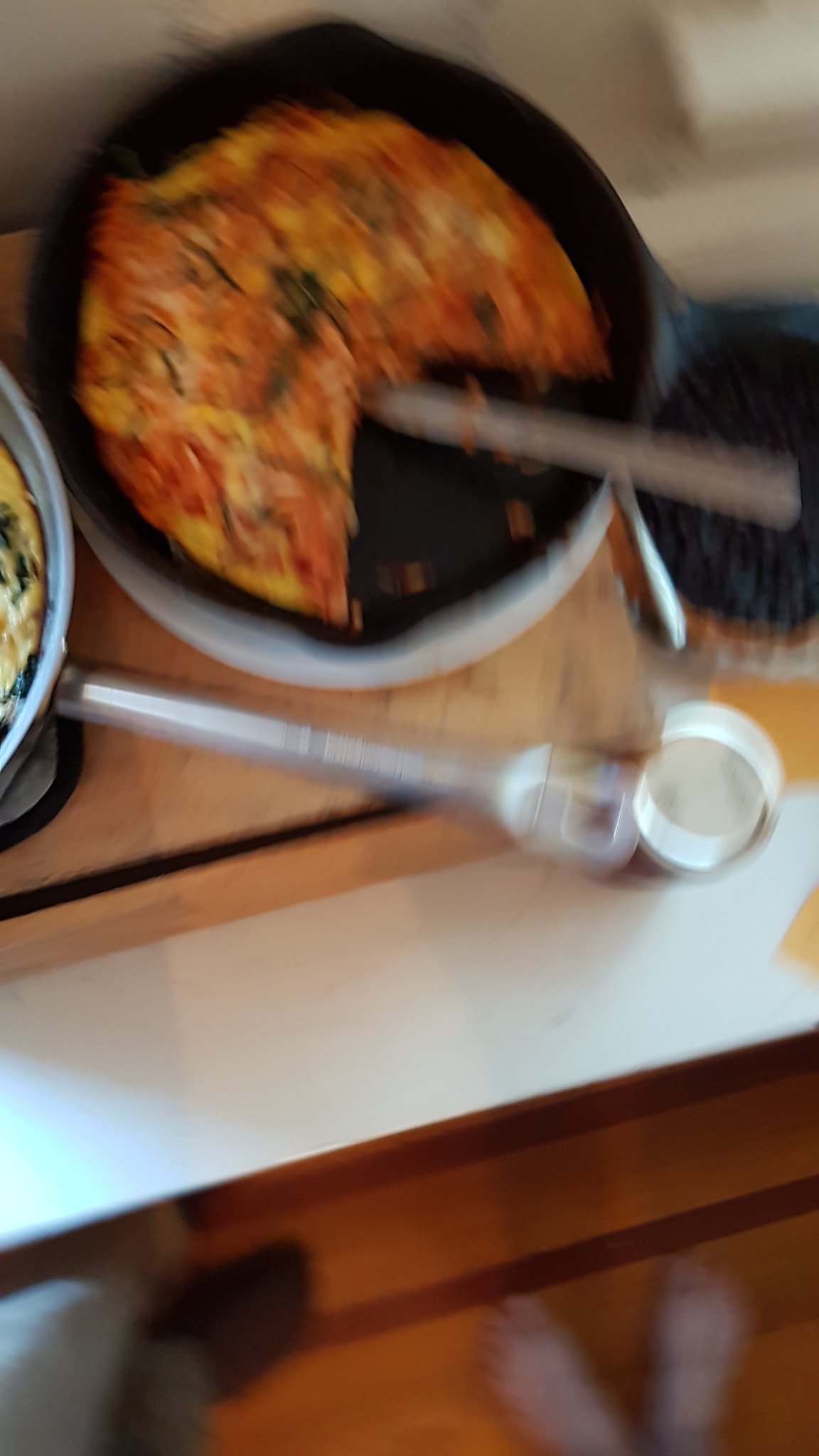In this overhead photograph, a scene unfolds on a white countertop that reveals an array of culinary elements. Dominating the top left of the frame is a round, black cast iron pot, which cradles a visually intriguing dish. The dish, possibly a tomato pie, features a noticeable triangular section removed, exposing layers of flat, sliced tomatoes. The surface of the pie is a mosaic of brown, green, and yellow hues, suggesting a perfect blend of baked ingredients and perhaps some herbs.

Emerging from the center of the cut-out triangle is a prominent brown rectangle, which adds a geometric contrast to the organic shapes within the pot. Supporting this pot is a white, circular dish, perfectly centered on a rustic wooden chopping block that has a distinctive black line at its base, marking a division. The chopping block itself rests securely on the pristine white countertop, creating a clean backdrop for the scene.

Beneath the expanse of the white countertop, the subtle warmth of a reddish-brown cabinet front peeks into view, adding a cozy touch to the composition. Adding to the culinary vignette, a silver garlic press lies diagonally just below the cast iron pot, suggesting recent use and hinting at the aromatic elements possibly woven into the dish. The careful arrangement and varied textures create an inviting and detailed snapshot of a kitchen moment.